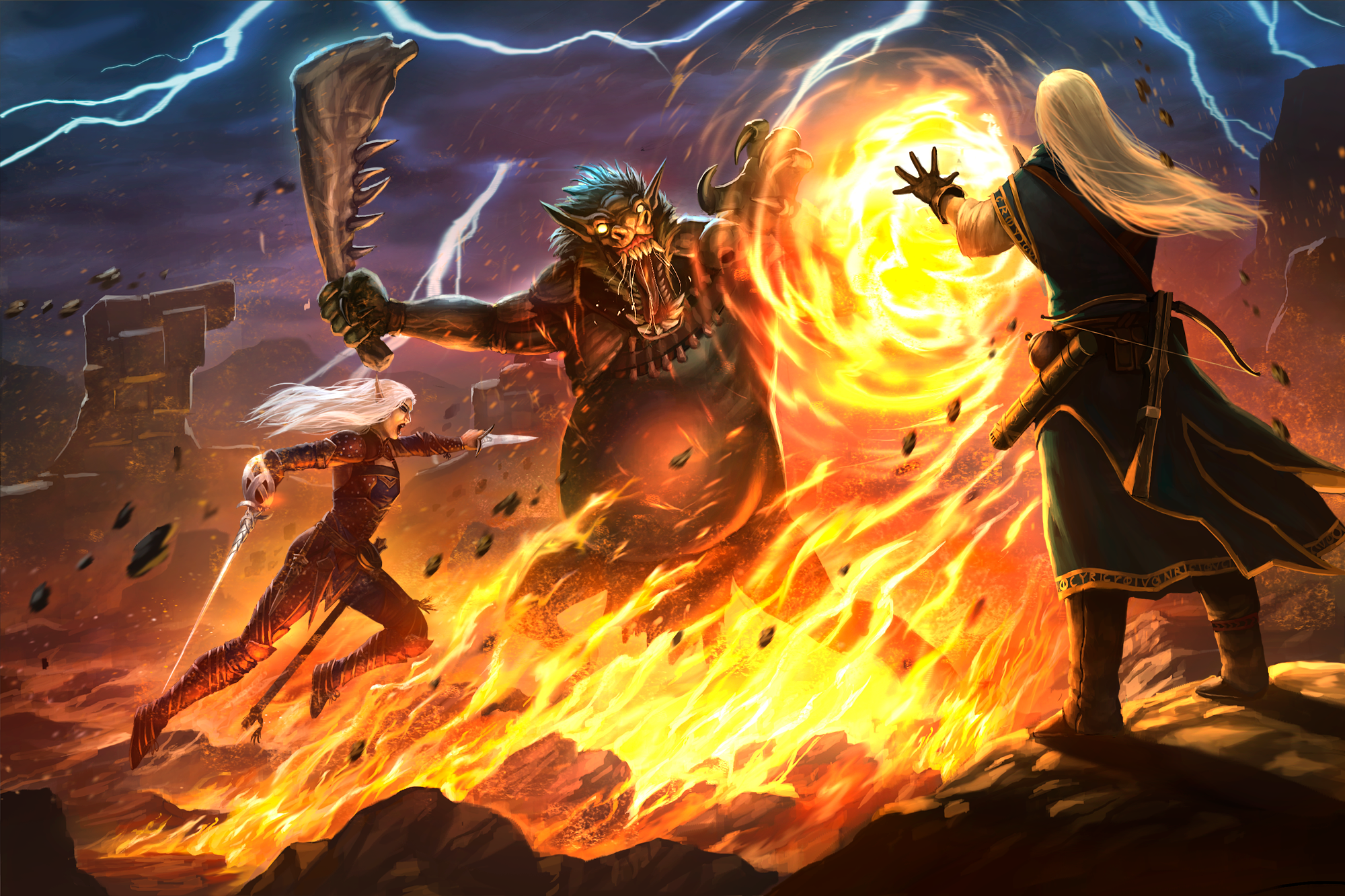The image depicts a dynamic and fantastical battle scene, likely from a game or a piece of fantasy artwork. The background is a dramatic blend of black and purple, lit by striking blue lightning bolts. In the center stands a menacing, werewolf-like creature with a large, protruding belly and wild hair. Its mouth gapes open to reveal spiky teeth, from which drool spills. The creature wields a fearsome weapon resembling a jagged jawbone or club with teeth embedded in it.

To the creature’s right, a male figure stands with his back turned, clad in a long dark green cape, brown boots, a white long-sleeve shirt, and black gloves. His long flowing white hair cascades down his back. He appears to be conjuring a fireball, poised to hurl it at the beast. Flames dance beneath his feet, contributing to the intensity of the scene.

On the creature’s left, a female elf with similar long, flowing white hair leaps into the fray. She brandishes a knife and a sword, aggressively advancing on the werewolf-like creature. Her face, unlike the fireball-throwing figure, is visible, marked by determination and fierce resolve. The scene is vividly animated, with elements of fire and magic intertwining against the tumultuous sky, heightening the sense of action and urgency in this mythical confrontation.